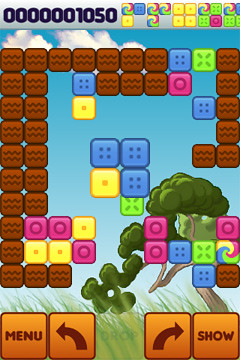The image is a vertically-oriented screenshot from a block-based video game, likely on a smartphone. The interface showcases a vibrant, animated outdoor scene with a blue sky and scattered white clouds. At the bottom of the screen are four light orange icons with dark brown text: "Menu," a left arrow, a right arrow, and "Show." The background at the bottom depicts green grass and a tree with a large, fluffy green top leaning towards the left, accompanied by a brown branch. The main game area is filled with an assortment of blocks in various colors, including brown, blue, yellow, green, and pink. Some of the blocks have numbers such as '4' in blue and '0' in pink, resembling dominoes, while others are blank. Additionally, black squares frame the top and sides of the screen. Overall, the blocks conglomerate to form a larger cube-like structure in the space available towards the top.